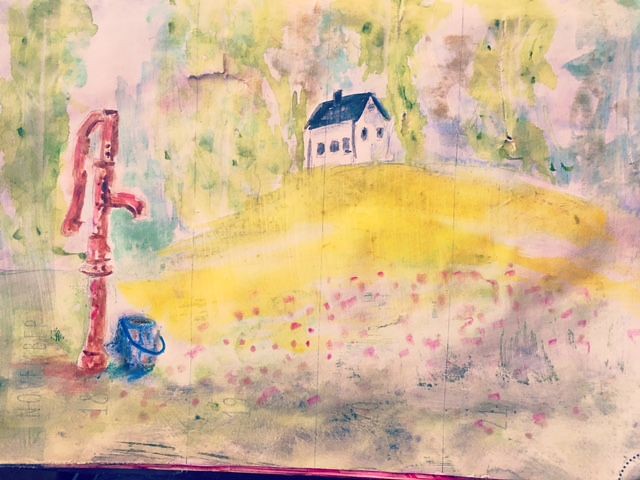The image depicts a colorful, child-like watercolor painting of a tranquil rural scene. Dominating the foreground, there's a vivid red, handheld water pump with a visible spigot and lever. Adjacent to the pump is a blue bucket placed on a lush-blueish green grassy area with small, scattered red flowers. The scene transitions into a yellow hill, suggesting dry grass or a sunlit field. Perched atop this hill is a distant, white house with a dark blue roof, outlined by some trees. The house is painted small to emphasize its distance. Numerous red dots pepper the image, likely meant to represent flowers or decorative elements. Additionally, partially legible black text is smeared on the bottom left, and numbers such as 18, 19, 20, and 21 are faintly visible. A distinct red horizontal line runs along the bottom, completing the vibrant and whimsical landscape.